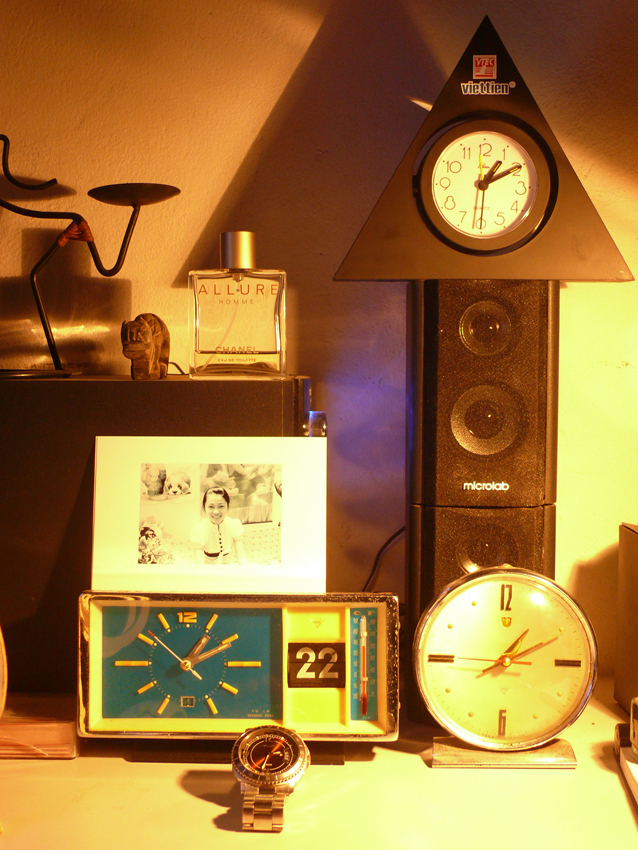In this detailed image, the focus is on various objects arranged on a table. The scene is closely zoomed in, showing only the lower portion of the table and the objects upon it. The table itself features a tannish-yellow color, with the right side appearing white due to the lighting.

At the center of the image, there is a wristwatch with a light brown strap. The watch face is dark brown with an orange dial. Directly above the watch is a rectangular clock featuring yellow lines and the number 12 at the top. To the right of this clock is another timepiece, circular in shape, with the number 12 and three brown lines marking the 3, 6, and 9 positions.

Further up in the image, a triangular-shaped clock is positioned above a speaker system. This triangular clock resembles an upward arrow and casts a shadow towards the left. Also visible is a stand holding a cologne bottle labeled "A-L-L-U-R-E," with another similar stand to its left.

The background of the image reveals a wall painted in a light tan color, which complements the overall warm tones of the scene.